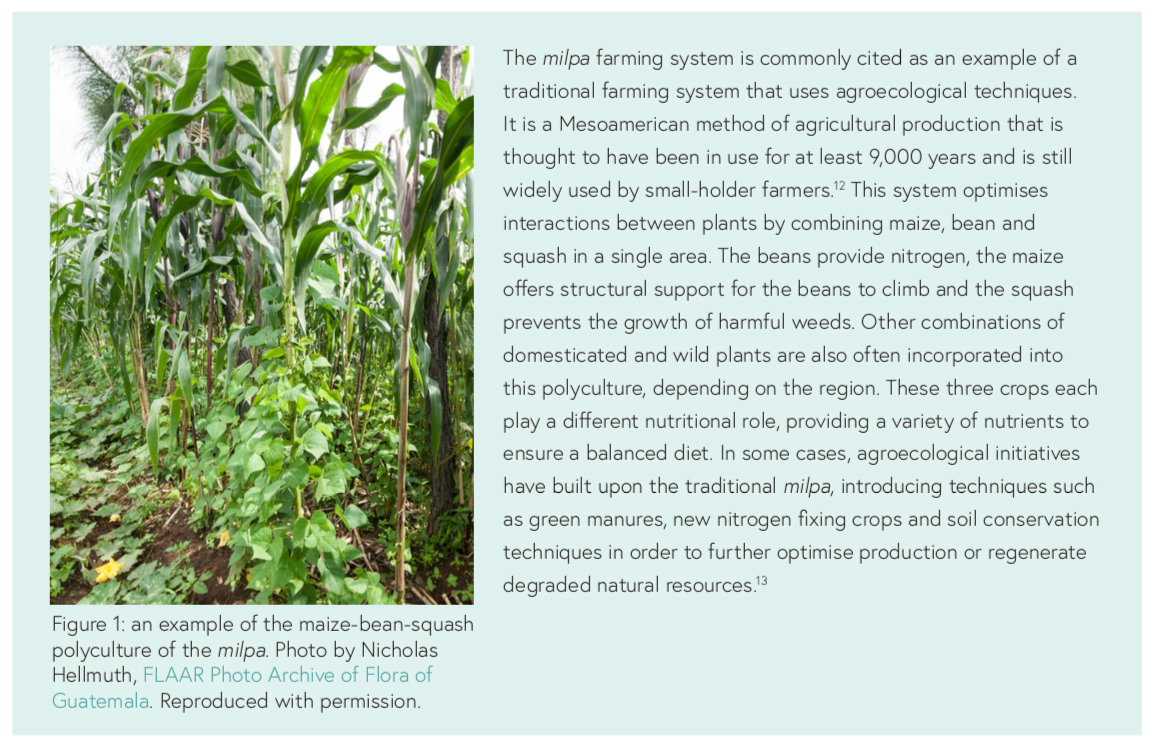This image depicts a vibrant garden featuring the traditional Mesoamerican Milpa farming system, illustrating a harmonious polyculture of maize, beans, and squash. The background is accentuated with a green hue, and to the left, a caption reads "Figure 1: An example of the maize, bean, squash polyculture of Milpa. Photo by Nicholas Helmuth, Flair Photo Archive of Flora of Guatemala, reproduced with permission." A detailed paragraph accompanies the photograph, explaining that the Milpa system, which has been in use for at least 9,000 years, is characterized by its agroecological techniques. This method enhances plant interactions: the maize provides structural support for climbing beans, the beans enrich the soil with nitrogen, and the squash spreads across the ground to prevent weed growth. This enduring method is still widely practiced by smallholder farmers today, often incorporating various combinations of domesticated and wild plants depending on regional traditions.